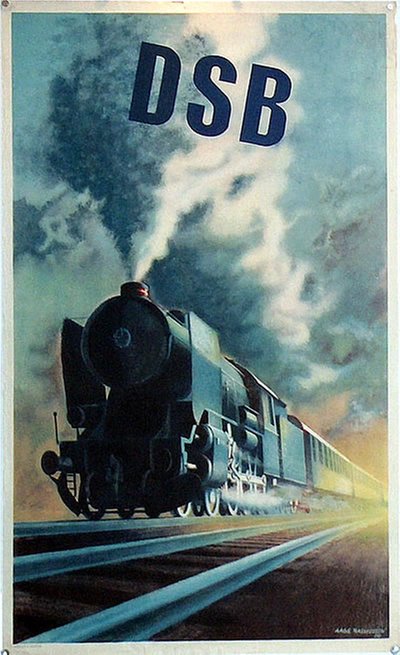The image is a detailed drawing or painting of an older steam locomotive train, likely intended to evoke a sense of nostalgia. The train is moving along a set of tracks that extend diagonally from the bottom left to near the bottom right of the image. The front of the train, which is much closer to the viewer and positioned towards the left-hand side, features a circular front design and is predominantly black, with parts of it in shadow, suggesting the sun is to the right and behind the train. The train has a prominently black first car with exposed wheels and red detailing in the smokestack area. 

Behind the first car, which likely holds coal, a series of train cars trail off into the distance towards the right side of the image. These trailing cars are mostly yellowish with windows lining their tops. Billowing from the front of the locomotive is a large cloud of white steam that darkens as it rises and spreads over the train. The backdrop includes a blue sky filled with clouds, transitioning to brownish or orangey tones near the horizon.

At the top of the image, above the steam cloud, are the capital letters “DSB” in a bold, dark blue font, suggesting a possible branding or title. The scene also includes an empty set of tracks in the foreground, highlighting the motion and direction of the train on the farther set of tracks.